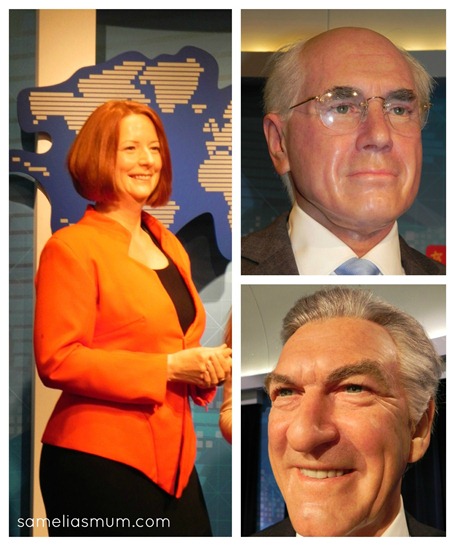This collage consists of three distinct photographs featuring different individuals. On the left, a photograph, occupying the entire left half of the collage, depicts a woman visible from her hips upwards. She wears a black skirt paired with a black shirt that has a low neckline and is topped with a blue blazer. Her short red hair frames her smiling face, which is turned slightly towards the right. In the bottom left corner of her photo, white text reads "semeliasmum.com." The right half of the collage is divided into two smaller photographs stacked vertically. The upper right photograph features a bald man with gray hair on the sides of his head, thin-framed glasses, and thick eyebrows. Donning a black business suit with a white shirt and a blue tie, his neutral expression is directed slightly off to the right. Below him, the bottom right photograph showcases another man, visible from the neck up, with silver hair combed back. He is wearing a dark jacket over a white shirt, smiling as he looks slightly off to the left. The background behind the woman features a blue wall with a design, hinting at a professional setting, likely reminiscent of a company website showcasing employees.